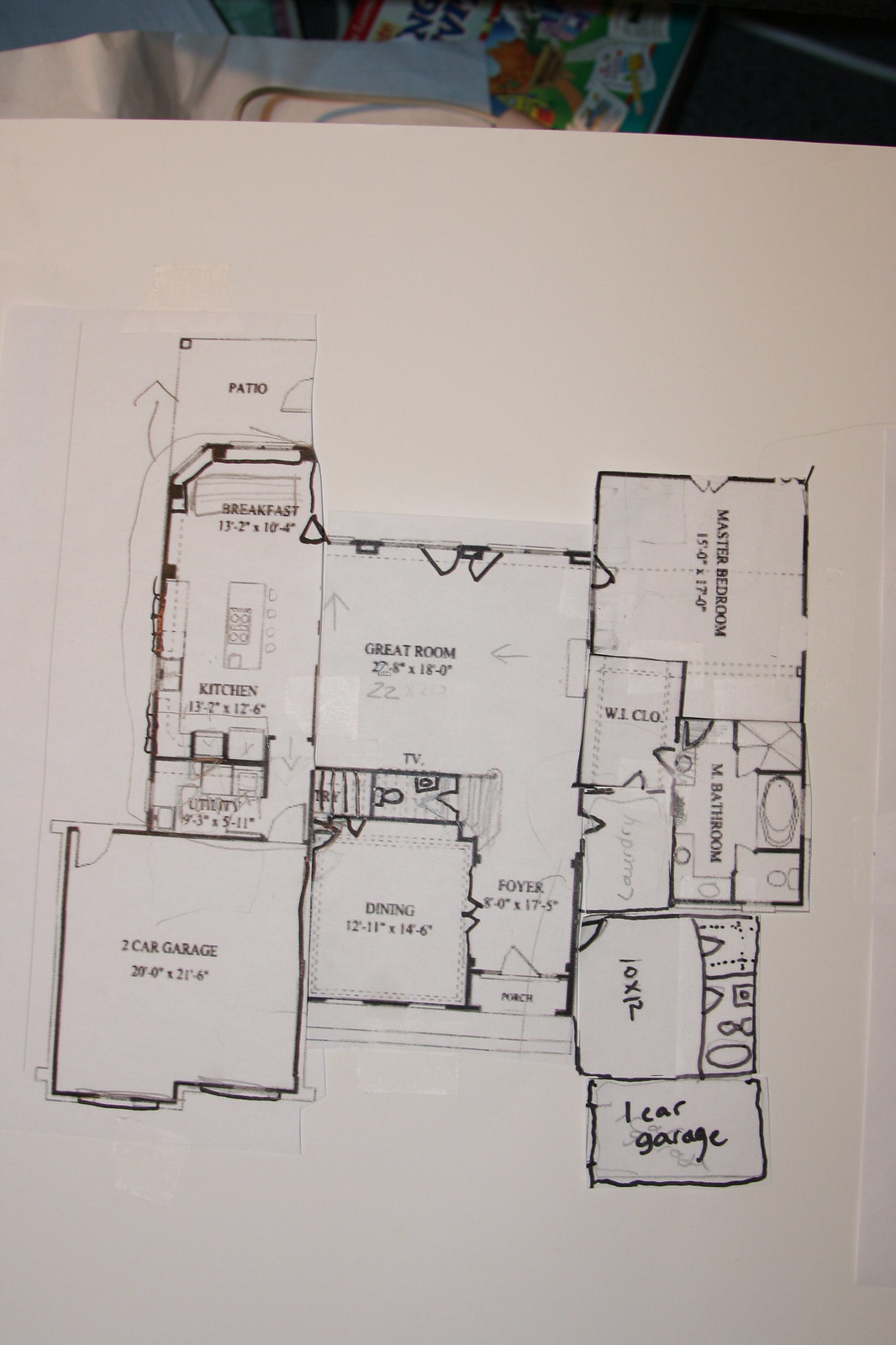The image presents a hand-drawn, pencil-and-pen floor plan diagram, affixed on top of a clean, white sheet of paper. The diagram appears to be meticulously cut out from another sheet, with precise outlines surrounding each room. Located on the bottom left corner of the plan is a two-car garage, directly adjacent to a dining room on its right. Above the two-car garage lies a sequential arrangement of a kitchen, a breakfast nook, and ultimately a patio area.

To the right of the dining room is a spacious great room, which is adjacent to a foyer. Directly to the right of the foyer is a designated 10 by 12 space, below which sits a one-car garage. Above this 10 by 12 space, the layout includes a master bathroom, a walk-in closet, and a conveniently placed laundry room. At the top of the diagram is the master bedroom, completing the floor plan.

Each room is labeled with small dimensions, carefully inscribed beneath the respective room names in black ink. Notably, the one-car garage, the 10 by 12 space, and an adjacent bathroom seem to be drawn in ink marker, standing out from the other elements. The rest of the plan’s annotations appear to be computer-generated text, complemented by roughly sketched outlines, creating a blend of digital and hand-drawn elements in the overall layout.